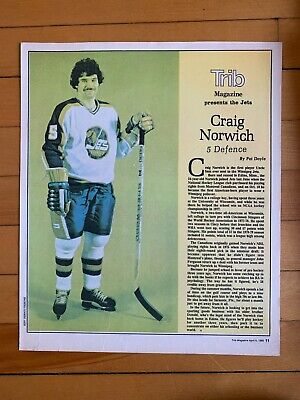A full-page magazine article on Craig Norwich, defense number five for the Winnipeg Jets, features a large photograph that spans from the top to the bottom of the page, bordered in white. Craig Norwich, with short curly black hair and a mustache, is smiling and posed in his complete hockey uniform. His jersey is primarily white with blue sleeves bordered in yellow, matching his blue pants with gray accents. He is equipped with long socks, ice skates, and a glove, holding a white hockey stick with a black handle and bottom in his left hand. The photo has a lime-green background. To the right of the image, a yellow column displays the text "Trib" in white at the top and "magazine" in black below, followed by "Craig Norwich, five defense." The main article begins beneath this text. The small black text and the page number 11 are found in the bottom right corner. The magazine is shown lying on a brown, slatted wooden surface.